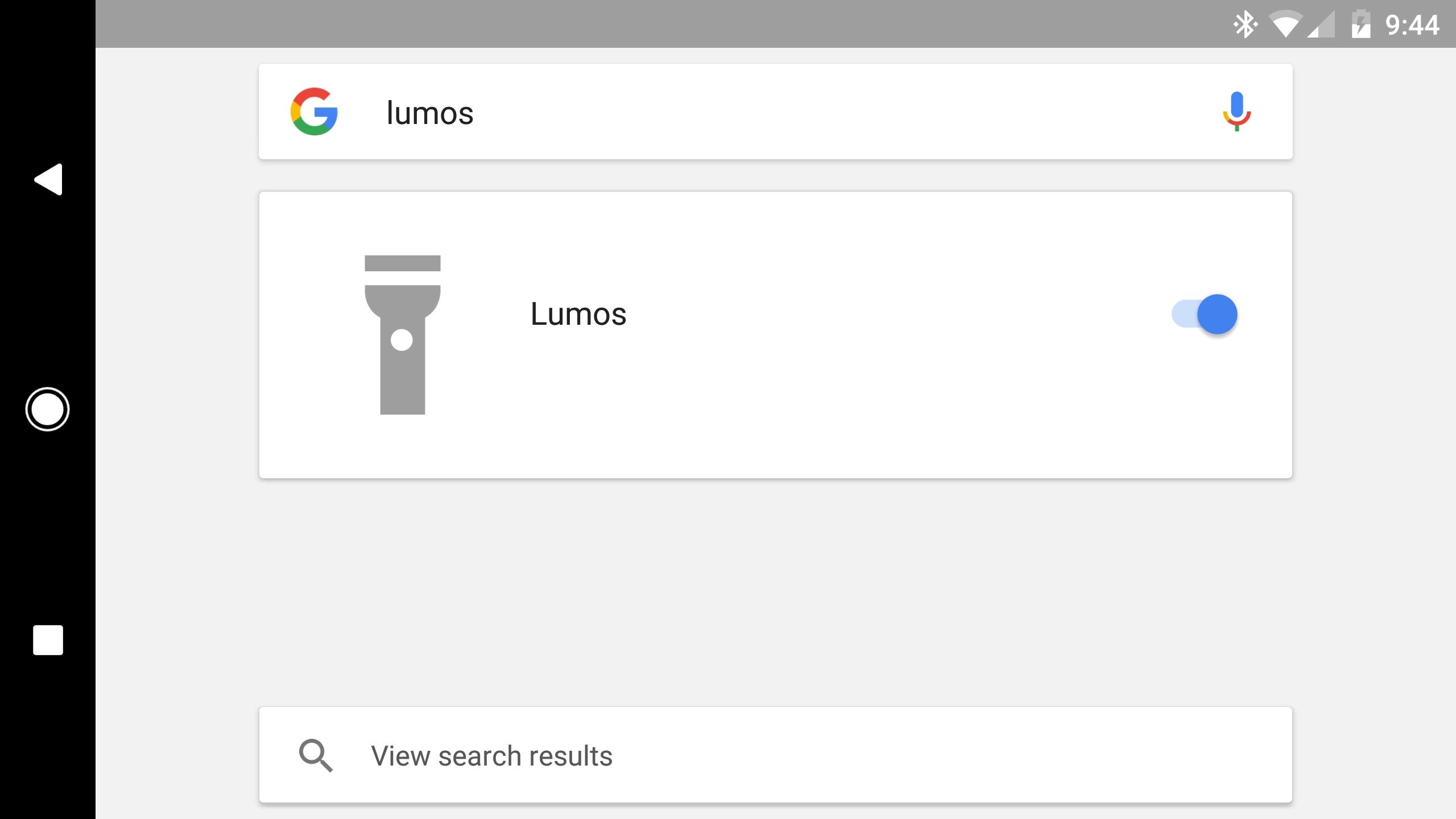This image appears to be a screenshot taken from a computer screen. The screen is displayed in a horizontal rectangular format, suggesting it is likely from a desktop or laptop computer. 

On the left side of the screen, there is a black vertical border containing three distinct white icons: a triangle pointing to the left at the top, a circle in the middle, and a square at the bottom. The top of the screen has a gray horizontal border that is mostly empty except for the right side, where there are several icons including a wedge, triangle, battery symbol, and a digital clock displaying the time as 9:44.

The central portion of the screen has a lighter gray background with a prominent horizontal search bar near the top. The search bar is white and features the Google logo, which is rainbow-colored, followed by the text "Lumos." To the right of this search box, there is a microphone icon that is blue and red.

Below the search bar, there is a larger white rectangle situated in the middle of the screen. On the left side of this rectangle is a gray flashlight icon pointing upward. Inside the rectangle, it also says "Lumos." Additionally, there is a slider button with a blue circle that can be toggled on or off.

At the bottom of the screen, there is a smaller white bar containing an hourglass icon on the left, next to the text "View Search Results." This detailed layout suggests the image could be from a user interface designed for searching or controlling specific functions on the computer.